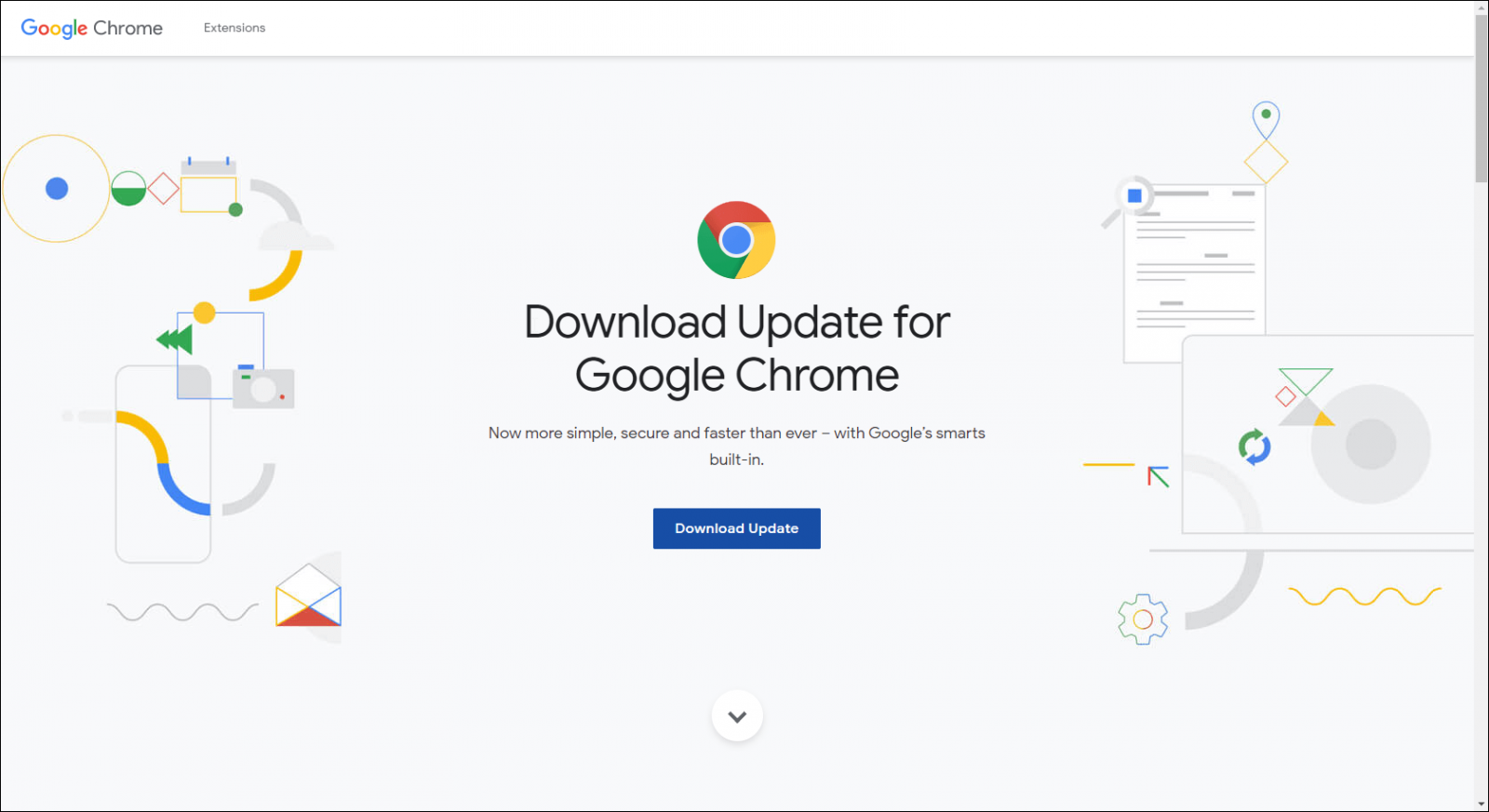This image is a cropped screenshot of the Google Chrome for desktop installation page. At the top left corner, the Google logo is displayed prominently, followed by the text "Chrome" in bold grey letters. Next to it on the right, there is text reading "Extensions," also in bold grey letters. The background of the page transitions into a grey color below these elements. 

Centrally positioned on the page is the Google Chrome logo. Directly beneath the logo, bold black text reads "Download Update for Google Chrome," conveying the page's primary call to action. Under this headline, there is a subtext in small grey letters that says, "Now more secure and faster than ever with Google smarts built-in," highlighting the benefits of the update. 

Below this, a large blue button, centrally aligned, features the text "Download Update" in bold white font. Additionally, at the very bottom center of the screenshot, there is an arrow pointing downward, further indicating the download link.

Decorative elements are present along the left and right sides of the screenshot. On the left, there are clipart illustrations, including envelopes, lines, circles, and calendars, depicted as simple line drawings. On the right side, similar clipart shows documents, shapes, and icons, adding a visual balance to the page layout.